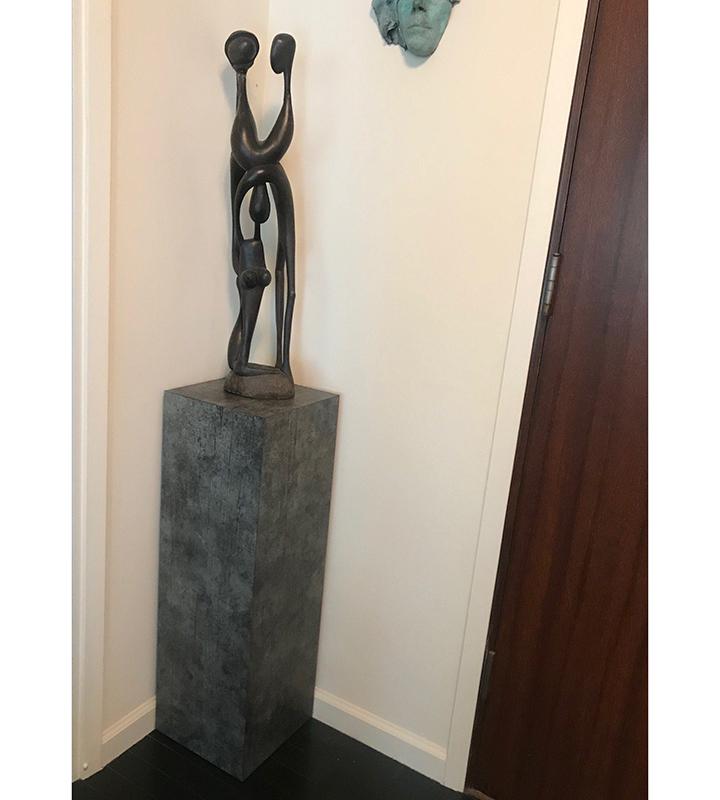This is a realistic photograph, vertically oriented, capturing the corner of a room. The room features white or cream-colored walls with white trim and a deep brown hardwood floor. On the right side of the image, there is a brown wooden door that appears to be made of walnut. In the top right section of the photograph, there is a partly visible green mask, resembling an ancient Greek bronze sculpture. Positioned at the center of the corner is a pedestal, approximately three feet high, and made of stone or a material painted to resemble gray marble. Atop this pedestal stands an abstract sculpture of three figures, likely representing a mother, father, and child. The sculpture features smooth, elongated shapes: the figures have small round heads and swooping lines for their bodies, arms, and legs, with the two taller figures appearing to hold hands in an arc-like shape, symbolizing unity and family.